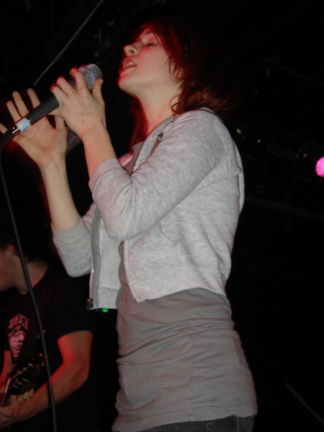In the image, a woman is captured singing with her eyes closed and head tilted upward. She holds a microphone in her left hand, with her right hand extended towards it but not touching. She wears a gray sweater, unzipped and pushed back off her wrists, over a longer grayish-brown shirt. The background is predominantly black with a few white and a notable pink dot near the center-right, possibly a light. In the bottom left, a man with dark hair, wearing a black T-shirt, is visible, seemingly playing a guitar, although only parts of his neck, ear, left arm, and shirt are discernible. The woman's fingernails are painted red, adding a touch of color to her grayscale attire, and the microphone cable extends downward from her left hand.